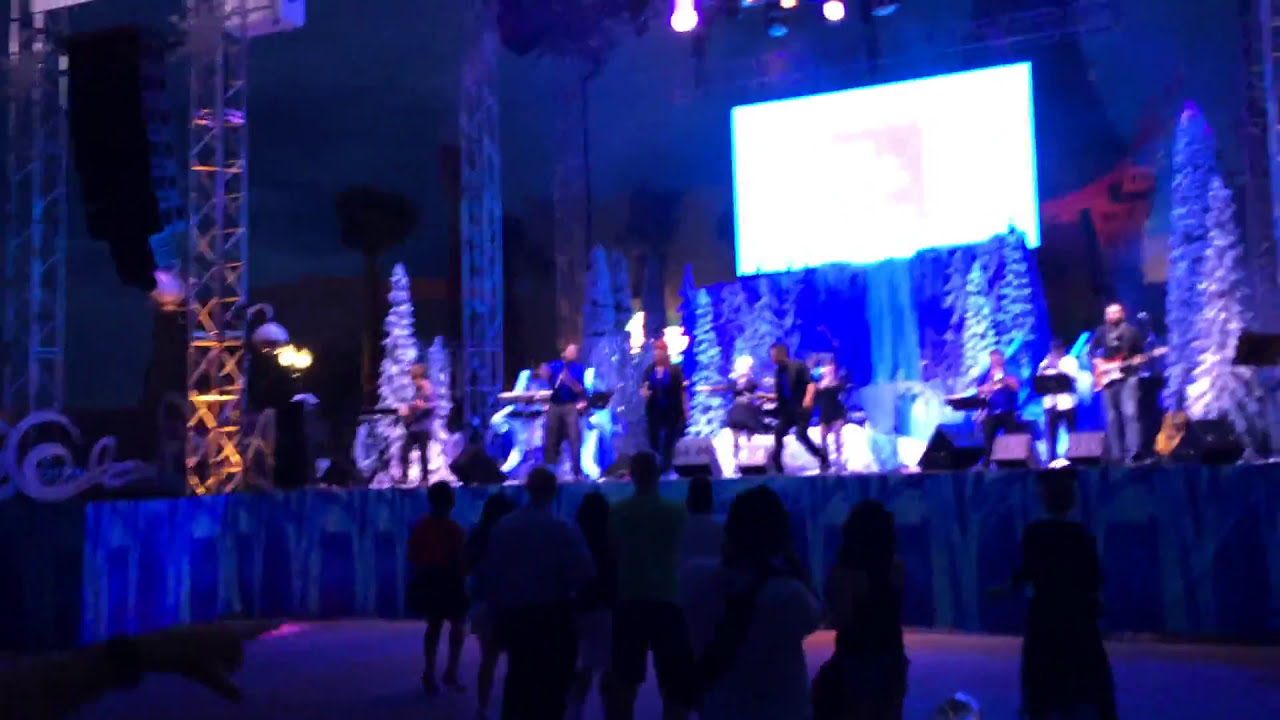The photograph depicts a dimly lit event space with a focus on a stage, which is bathed in a blue hue from the stage lights. In the foreground, there is a shadowed audience of about ten people facing the stage. The stage apron features a distinct blue pattern, and towards the left, metallic scaffolding supports the lighting rigs. On stage, we see an eight-piece band, some members playing instruments like guitars and keyboards while others appear to be singing. The backdrop of the stage creates a winter scene with artificial pine trees covered in snow, and a large white display screen is positioned high above the center-right of the stage. The overall composition is a bit blurry, adding to the ambient and immersive feel of the performance.